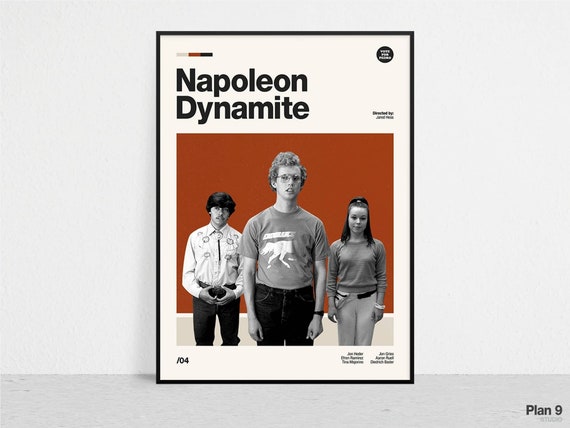This image features a framed poster of "Napoleon Dynamite," leaning against a light gray wall with a dark gray floor, possibly standing on a table or the floor itself. The poster, encased in a thin black border, has an off-white background with the title "Napoleon Dynamite" written in black at the top, accompanied by small symbols in the top left and right corners. Below the title, there is a dark orange square containing a photo of the three main characters from the movie. The central figure is a young man in a light-colored t-shirt and long dark pants, his hands hanging at his sides with a dark watch on his left wrist. To his left stands another man in a white shirt and dark pants with short dark hair, and to his right is a white woman with long dark hair, wearing a light-colored, long-sleeved knit top. At the bottom of the orange square, the background turns a grayish hue. On the very bottom right of the poster, within the gray floor area, the words "Plan 9" are visible. There is also a faint dash and the numeral zero-four (04) followed by some unreadable text beneath the photo.